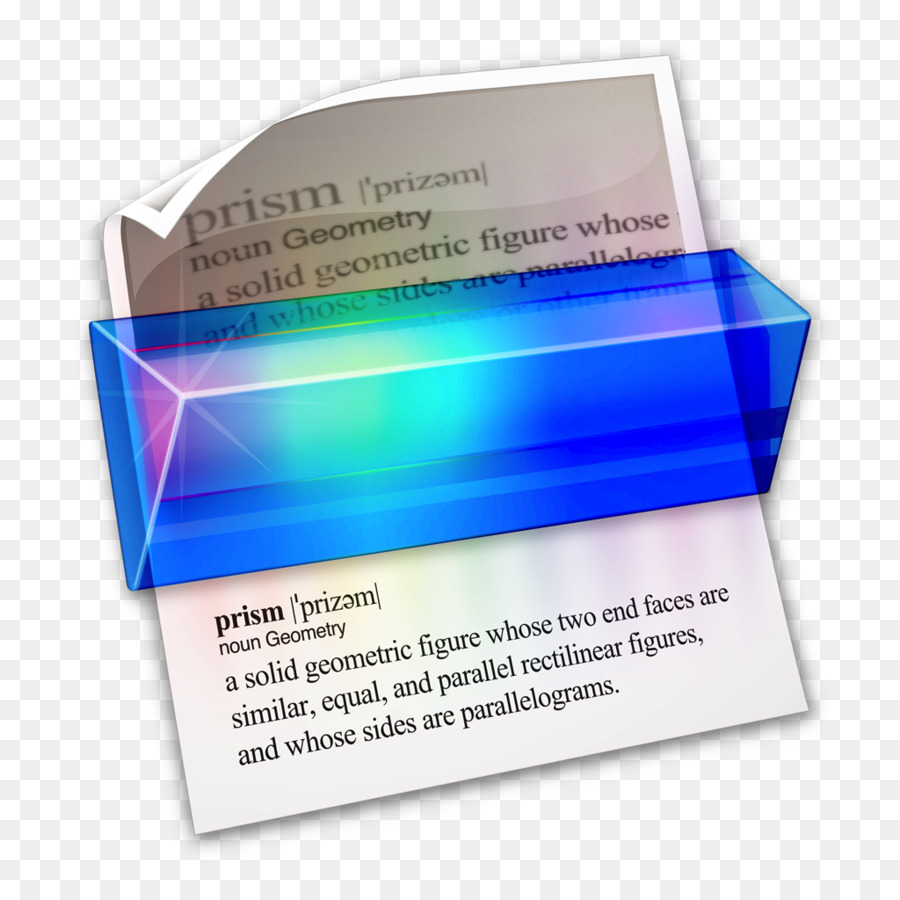The image depicts a curved sheet of paper set against a small, checkered background of alternating light blue or gray and white squares. Dominating the center of the paper is a visually striking, large, blue prism that showcases hues of turquoise, magenta, and purple, with a mild star shine and two rainbow lines emanating from the top angle. The paper features the word "prism" twice, each time followed by its pronunciation and the label "noun, geometry." The definition is interrupted by the prism but repeats at the bottom, stating, "A solid geometric figure whose two end faces are similar, equal, and parallel rectilinear figures, and whose sides are parallelograms." The text on the paper is in black, enhancing the contrast with the bright, reflective prism.